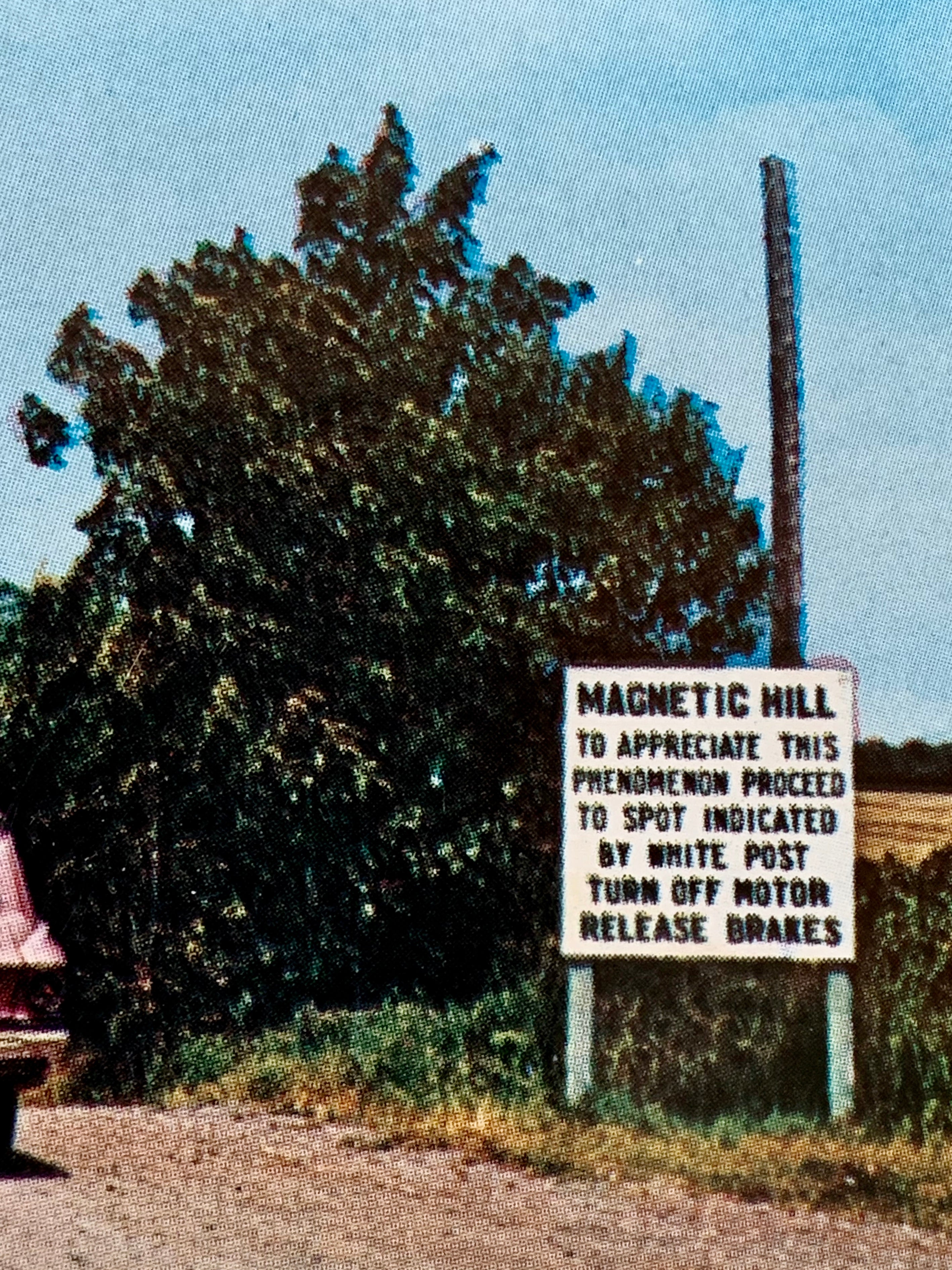This grainy, low-definition image, which seems to straddle the line between a photograph and a painting, is taller than it is wide. Dominating the scene is a large, dark green bush situated centrally. To the right of the bush, a tall, grayish-black pole or tower extends upward. In the background, the sky is a clear blue, suggesting a sunny day. A white sign on wooden stilts stands prominently near the bush. The sign reads: "Magnetic Hill. To appreciate this phenomenon, proceed to spot indicated by white post, turn off motor, release brakes." In the foreground, a gravel or dirt road stretches out in front of the bush and sign, bordered by patches of green and brown grass. Towards the bottom left corner of the image, a small, barely visible sliver of a pink vehicle—most likely a car—peeks into view. The scene is framed by a slight glimpse of a field with yellowish grass or wheat, adding depth to the composition.